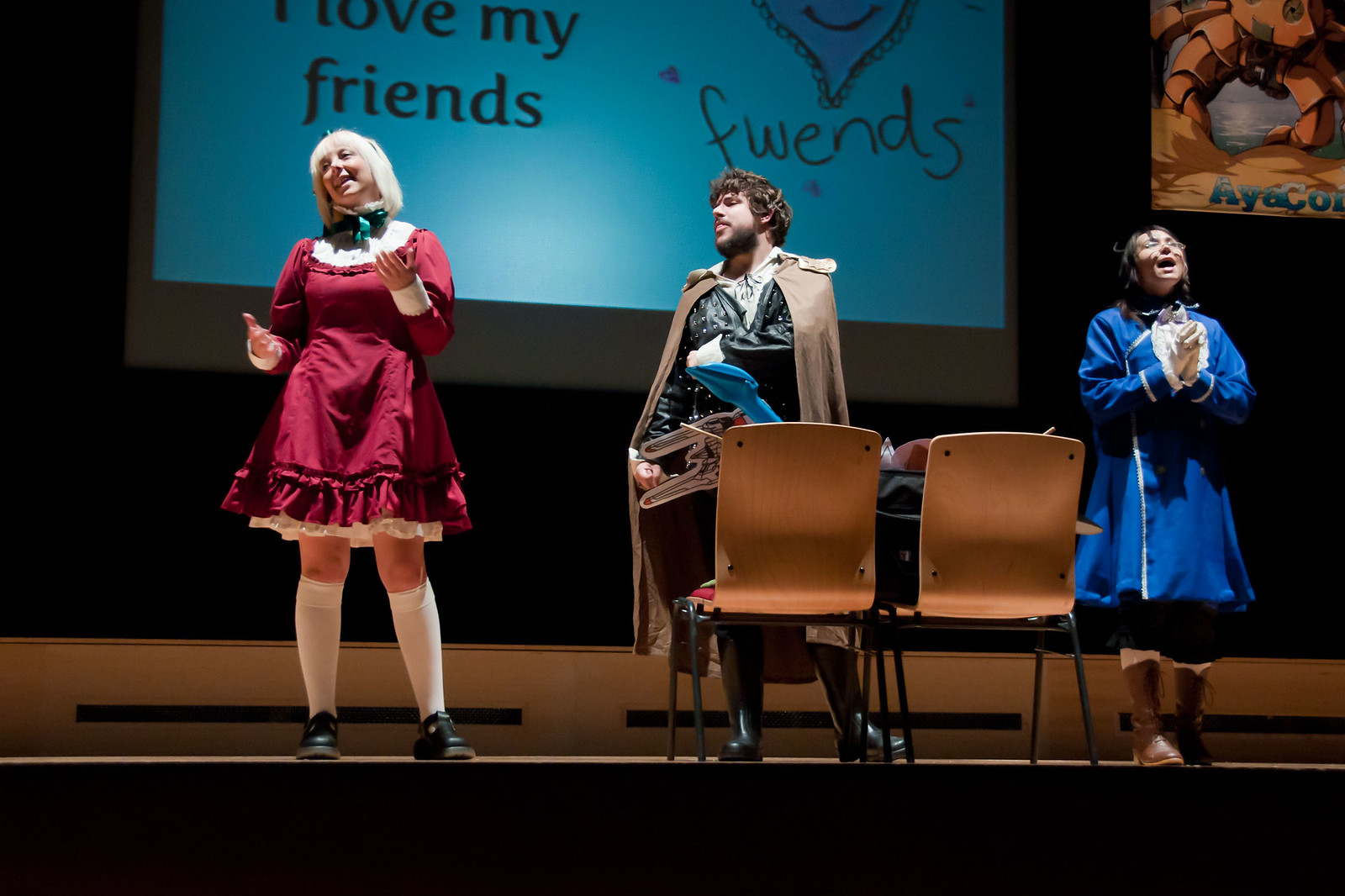On a dimly lit stage, three young performers are captured in the midst of what seems to be a high school play or production. Centered behind them, a large projection screen displays the whimsical message, "I LOVE MY FRIENDS," embellished with a heart doodle and the word "FWENDS" spelled in a playful manner.

On the left, a young woman with short white-blonde hair stands out in a vintage-inspired, short red dress with a frilly collar and a distinctive green bow. Her knee-high socks and poised demeanor add to her character's charm. In the middle, a young man with shaggy brown hair and a medium-length beard dons a black leather shirt under a brown cloak. He holds a mysterious prop and gazes thoughtfully to the left. On the right, a young woman in a striking long blue dress with black earrings and glasses commands attention as she looks upward, seemingly singing with passion. Her hands are clasped in front of her, adding to the intensity of her performance. 

In front of the trio, two chairs face inward, their surfaces possibly holding more props that blend into the scene, enhancing the theatrical ambiance. These are the only figures illuminated in the otherwise darkened stage, creating a captivating tableau.